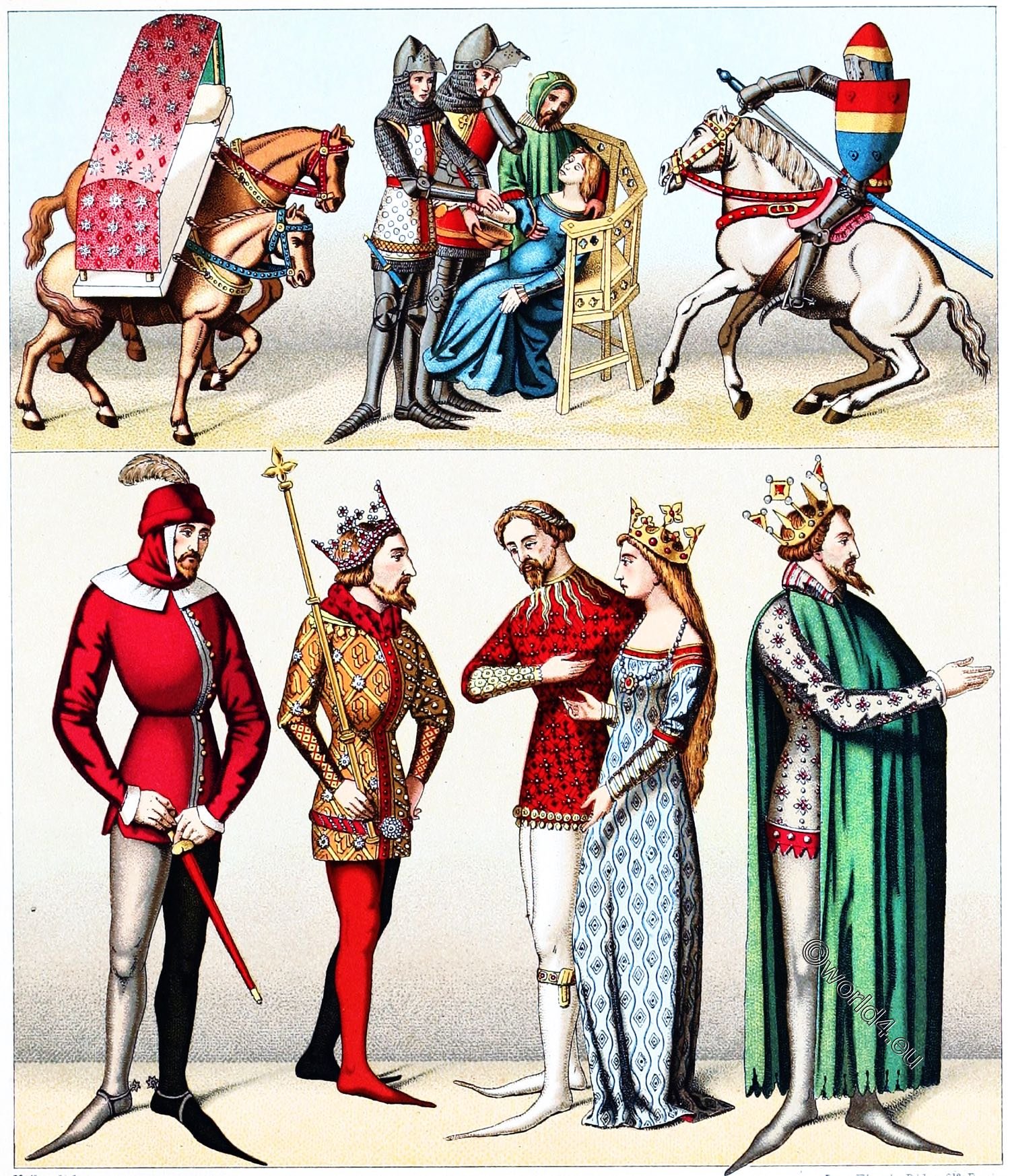This image is a detailed drawing reminiscent of Victorian times, possibly later, attempting to imitate or evoke medieval style elements. The artwork is divided into two distinct sections, the top and the bottom.

In the upper, smaller section, there is a pregnant woman dressed in a blue gown seated on a chair, attended by a variety of figures. To her left, two horses jointly carry an uncovered bed, appearing somewhat like a coffin with a pillow inside. This unusual detail contrasts with the surrounding elements. Standing next to the woman are two knights in traditional armor, one holding a brown bowl, and a monk in a green robe. On the far right, a warrior clad in armor and wielding a sword, rides a white horse, with a shield adorned in red, yellow, and blue.

The bottom section showcases a larger scene with five figures dressed in regal medieval attire. On the left, a man in red tights stands beside a woman wearing a gold crown. To the right, three men, distinguished by their crowns, suggest royalty; the central figure in red with a crown and a cross may signify a king. Another crowned male figure wears a lion-emblazoned robe, indicating high nobility, yet lacks the symbolic cross sword held by the presumed king. Together, these figures evoke a courtly tableau, rich in historical costume and significance.